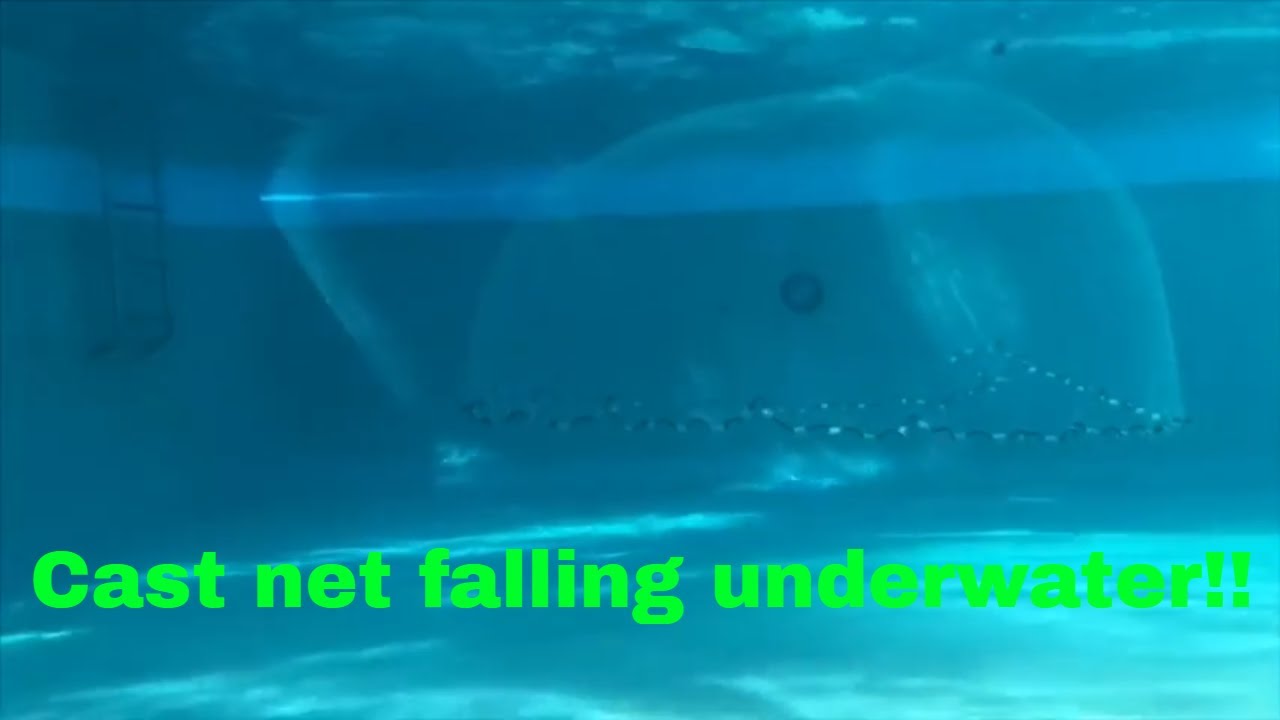This underwater scene, likely taken in a pool, captures a moment beneath the surface in varying shades of turquoise, darkening as it ascends. Prominently featured on the left side is a metal ladder extending halfway down the pool wall. An underwater light, possibly illuminated by sunlight filtering through, is visible to the right of the ladder. A faint, semi-circular cast net extends from the top to the bottom, partially obscured but discernible by its dark border adorned with multiple white circles. The scene is framed under a fluorescent green caption reading "Cast net falling underwater," with two exclamation points, adding a vivid, textual element to the image.